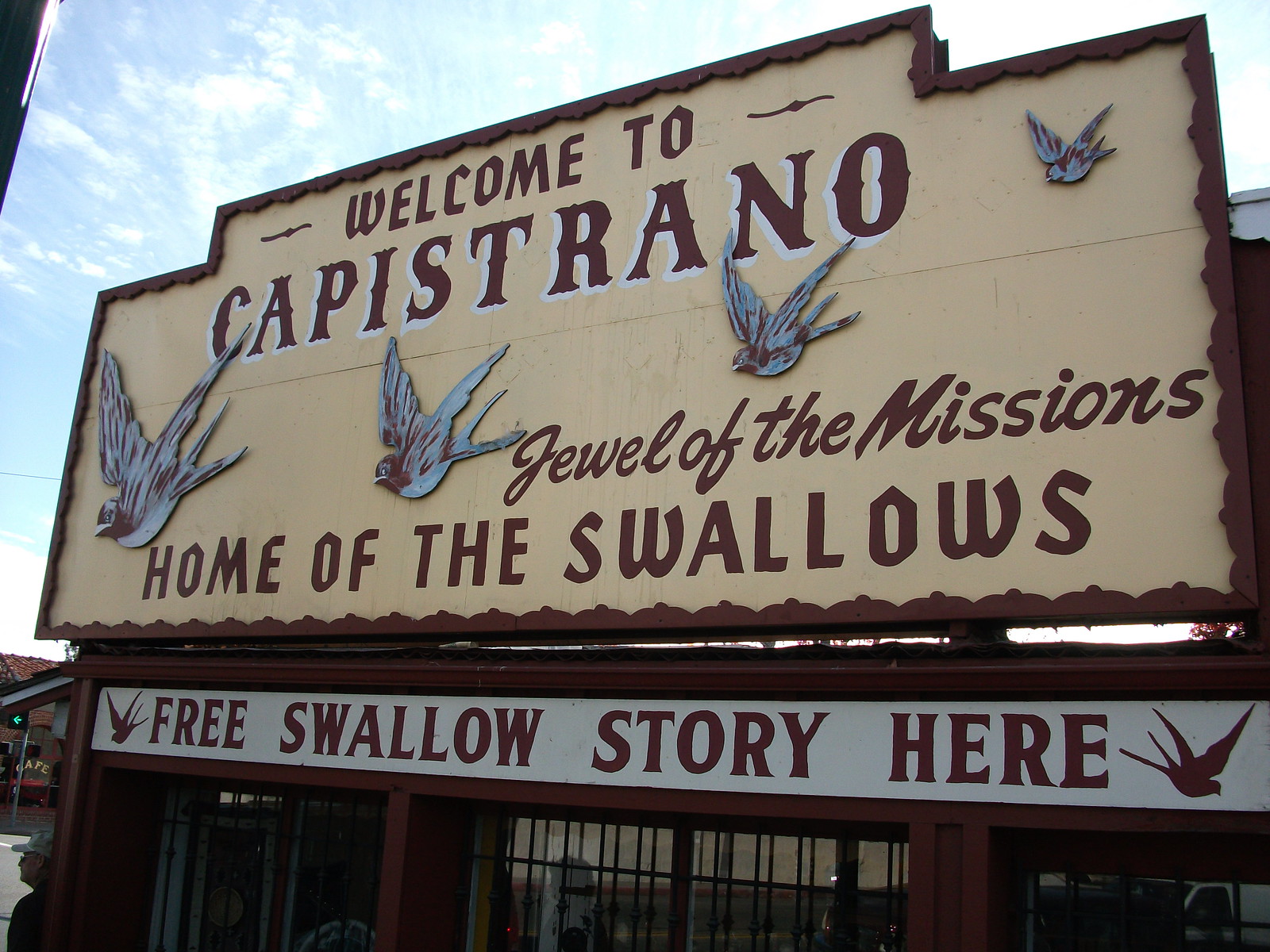The image depicts a large rectangular outdoor sign mounted on a dark wood building, basking in sunny weather with some clouds punctuating the blue sky. The sign, designed with a yellow-tan background and brown border, warmly welcomes visitors to Capistrano. It reads "Welcome to Capistrano" in a classic, cowboy saloon-style font, followed by "Jewel of the Missions" in cursive and "Home of the Swallows" in a Gothic or Old English script. Four swallows are illustrated on the sign, arranged from largest to smallest, flying from left to right. Below the main message, a banner in standard font announces "Free Swallow Story Here," flanked by images of swallows on each side. The establishment's windows are partially visible, but no people can be clearly seen, apart from possibly a distant figure. The sign's intricate detailing and historical emphasis suggest it caters to tourists, inviting them to explore the rich heritage and unique charm of Capistrano.